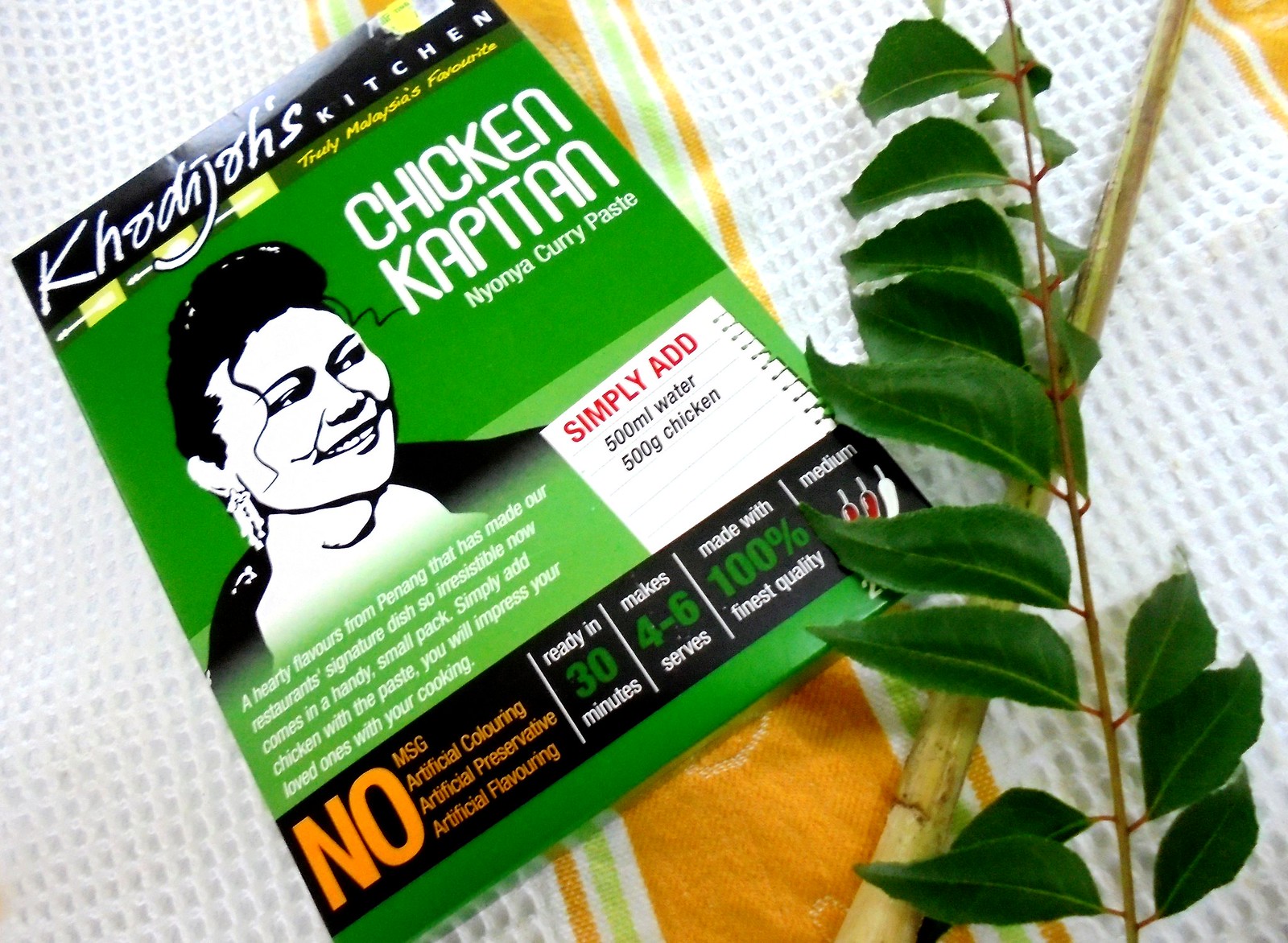The image features a green package labeled "Khodijah’s Kitchen" with a black bar at the top displaying the name in a special white font. Below it, the text "Truly Malaysia's Favorite" is written in yellow. The package prominently features a black-and-white illustration of a woman wearing earrings and a black jacket. The product is identified as "Chicken Kapitan Nyonya Curry Paste." The description highlights the hearty flavors from Penang, a signature dish from the restaurant, now available in a convenient small pack. The packaging instructs to simply add 500 milliliters of water and 500 grams of chicken, promising to impress loved ones. It emphasizes being free from MSG, artificial coloring, preservatives, and flavoring, with a preparation time of 30 minutes, serving 4-6 people, and being of medium heat with chili pepper icons. The package rests on a white linen towel with orange and green stripes, accompanied by a piece of bamboo and a stalk with green leaves.